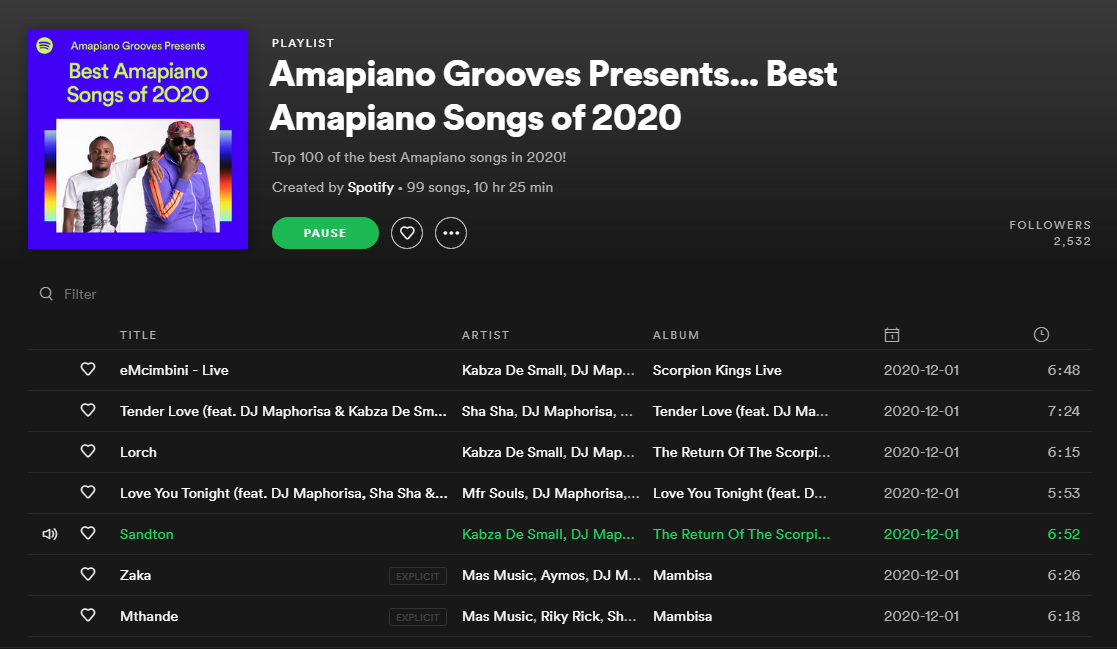Screenshot of a Spotify playlist titled "Emma Piano Grooves Presents Best Emma Piano Songs of 2020." The playlist title and details are displayed in white text against a black background. To the right of the title is the album cover, featuring a dark purple background with lime green text that reads "Emma Piano Grooves Presents Best Emma Piano Songs of 2020." The cover art depicts two Black musicians standing against a white backdrop. The musician on the right wears a purple tracksuit with orange stripes down the sleeves and an orange bandana.

Underneath the title is a green pause button. This playlist is curated by Spotify and contains 99 songs, with a total playtime of approximately 10 hours and 25 minutes. The interface shows a list of songs with columns for the title, artist, and album.

The first song listed is "E.M. Simbini Live" by Kabsa Dismal and DJ Map, from the album "Scorpion Kings Live." Five rows down, a song titled "San Tan" is highlighted in green text, distinct from the other entries, which are in white. "San Tan" is also by Kabsa Dismal and DJ Map, from the album "The Return of the Scorpio," and has a duration of 6 minutes and 52 seconds.